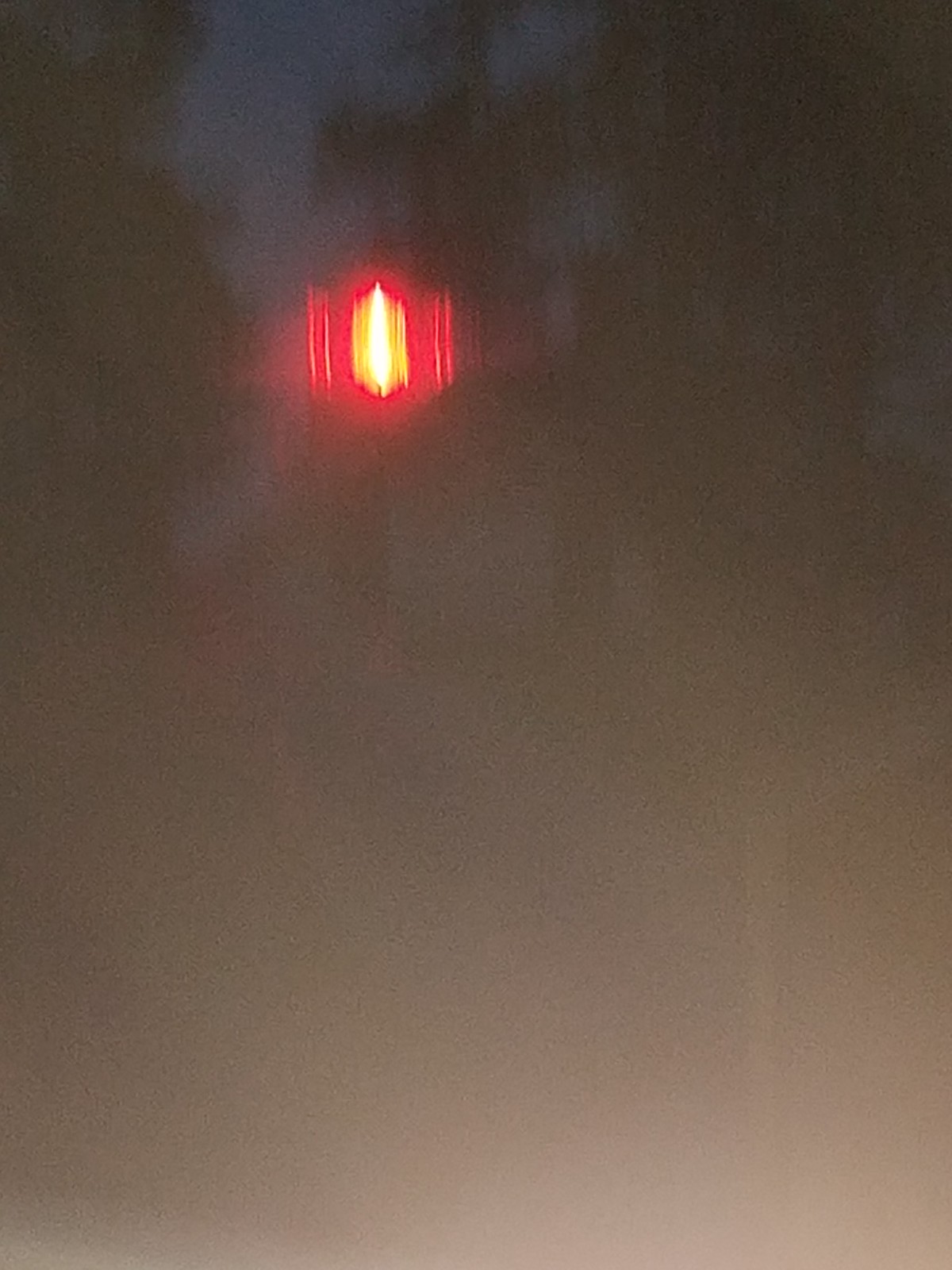This image is a very blurry photograph taken in a dimly lit outdoor setting, roughly one and a half times as tall as it is wide. The bottom two-thirds of the image is an indistinct blur, likely due to a thumb partially covering the lens, showing the light brown and dark brown tones of Caucasian skin. The scene appears to be captured just after sunset, with the sky transitioning to darkness. The upper portion of the image features the silhouettes of tree canopies against a twilight sky. In the top left and right corners, there are black outlines of trees. A prominent red and yellow light source, possibly a street light, is visible about 40% from the left and a third down the image, creating a glowing glare that stretches due to motion blur. Towards the bottom of the photo, there's a white glow, which could be an additional light source or the result of overexposure from the light brown blur. The overall scene gives an impression of looking up through the trees at a glowing light in a darkening sky.